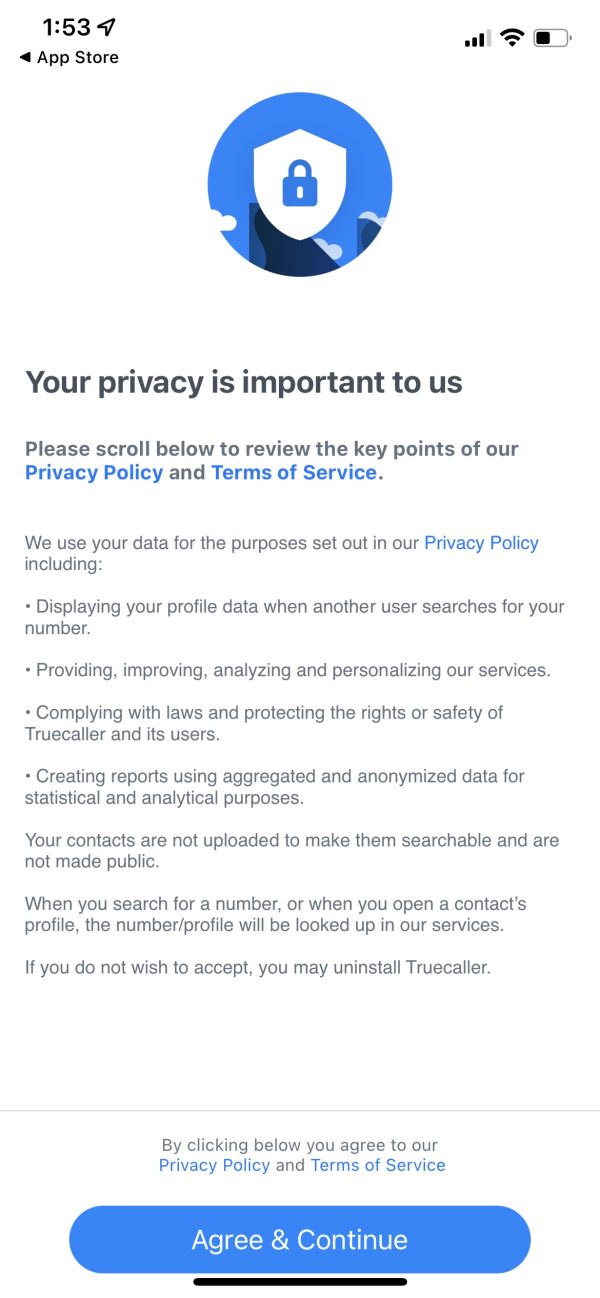The image appears to be a screenshot of a mobile phone display with a white background and various text elements in black and blue fonts. On the left side, there is a black number "153" with an arrow pointing to the right. Below that, with an arrow pointing to the left, it says "App Store". To the right, icons for Wi-Fi and battery status are visible.

In the center of the image, there's a prominent blue circle containing a white badge with a blue lock and a gray mountainous graphic underneath. Below this graphic, the text "Your privacy is important to us" is written in black font. Smaller black text follows, stating, "Please scroll below to review the key points of our," with "privacy policy" and "terms of service" highlighted in blue.

The subsequent text outlines the key points of the privacy policy:
- "We use your data for the purposes set out in our privacy policy, including:" 
  - "Dot: Display your privacy data when another user searches for your number."
  - "Dot: Providing, improving, analyzing, and personalizing our services."
  - "Dot: Complying with laws and protecting the rights or safety of Truecaller and its users."
  - "Dot: Creating reports using aggregated and anonymized data for statistical and analytical purposes."
- "Your contacts are not uploaded to make them searchable and are not made public."
- "When you search for a number or open a contact's profile, the number/profile will be looked up in our services."
- "If you do not wish to accept, you may uninstall Truecaller."

At the bottom, after a gray line spacer, there is a statement in black font: "By clicking below you agree to our," followed by "privacy policy" and "terms of service" in blue. At the very bottom, a blue circle with white text inside says "Agree and Continue," and a thin black horizontal line is beneath it.

Overall, the image serves to inform users about the privacy policy and terms of service, culminating in an action button to agree and continue.